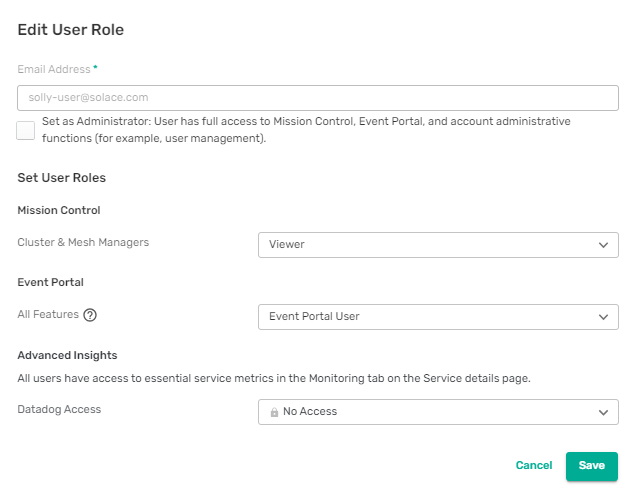The image shows a web page interface on a white background, designed for user role management but providing no indication of the platform, whether PC or mobile device. At the top, in bold black text, the heading reads "Edit User Role." Directly underneath, it says "Email Address" in light gray with a blue asterisk indicating a required field. A horizontal rectangle box contains an email address, "soli-user@solace.com."

Below this, there is a checkbox option labeled "Set as Administrator: User has full access to Mission Control, Event Portal, and account administrative functions (e.g., user management)." 

Further down, users can set specific roles under "Mission Control," with options for "Cluster" and "Mesh Managers" displayed in lighter font. There is a dropdown menu next to a rectangle labeled "Viewer." 

Under the "Event Portal" section, marked by a question: "All Features?", another rectangle specifies "Event Portal User" with a dropdown menu icon.

In the "Advanced Insights" section, a statement clarifies that all users have access to essential service metrics in the monitoring lab on the service details page. The user can set "Data Dog Access" through a dropdown menu currently showing "No Access."

At the bottom, there are two buttons: a green "Cancel" button, and a green button with white text that reads "Save."